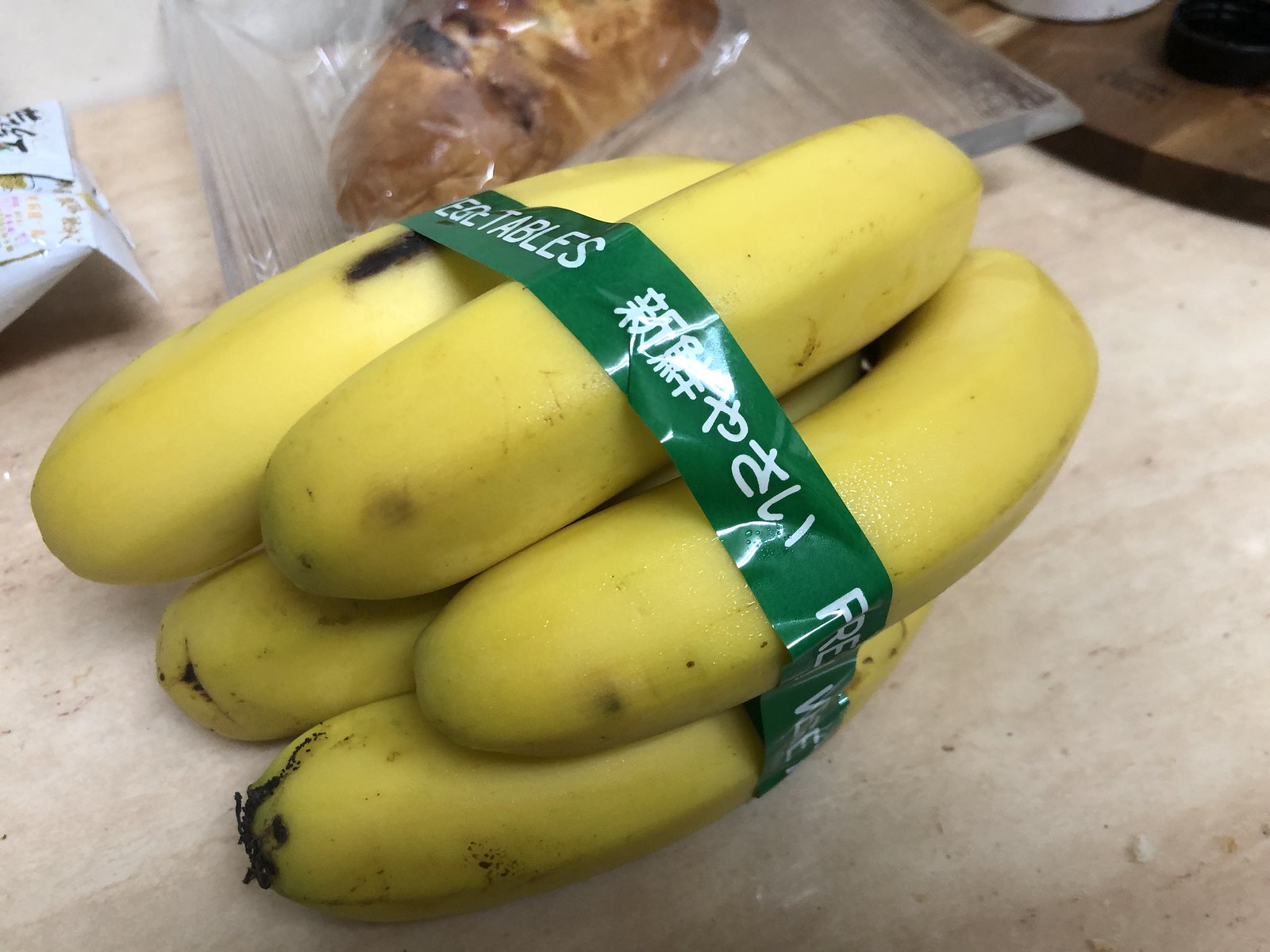This photograph captures a bunch of perfectly ripe, stubby bananas, distinct from the standard pointy-ended variety, as they feature rounded ends and have some dark spots indicating minor bruising. The bananas are grouped together with a green band, bearing both Chinese (possibly Japanese) writing and English text that partially reads "TABLES," likely part of "FRESH VEGETABLES." The bananas rest on a slightly dirty, light-colored wooden table. In the background, there is a glass dish containing a bread roll wrapped in plastic, a small bag of chips, and a glimpsed white package. A dark wood cutting board is visible in the upper right corner, and the seat of a chair with the bottom of a white jar or can on it is seen near the bottom edge of the frame.